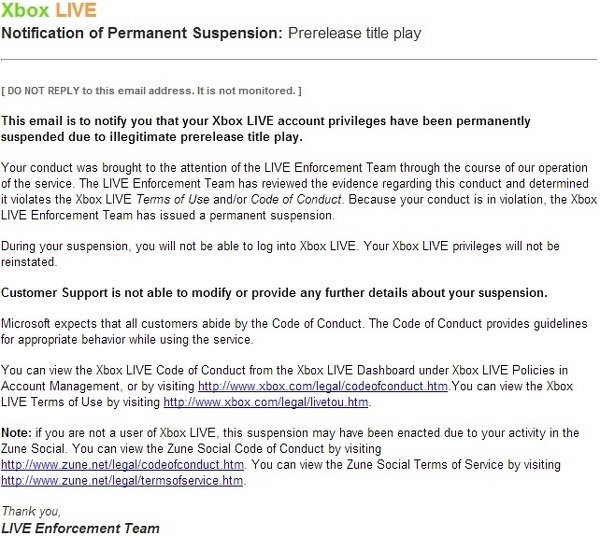The image is a notification from Xbox Live, detailing a permanent suspension of account privileges due to illegitimate pre-release title play. 

In the header, the word "Xbox" appears in green lettering with a yellow background, while "Live" is displayed in gold. The notification emphasizes that recipients should not reply to the email as it is not monitored. The email explains that the Xbox Live enforcement team identified and reviewed evidence of conduct that violated the Xbox Live Terms of Use and Code of Conduct. Consequently, the account has been permanently suspended, prohibiting access to Xbox Live. The email further states that customer support cannot modify or provide additional details regarding the suspension. 

Microsoft's expectation is that all users adhere to the Code of Conduct, which outlines appropriate behavior while using the service. Users are directed to view the Code of Conduct and Terms of Use through the Xbox Live dashboard under account management, or by visiting the specified website. The notification also mentions that non-Xbox Live users may have been suspended due to actions in the Zune social service, and provides a link to the Zune social code of conduct. The email concludes with a note of thanks from the Xbox Live enforcement team.